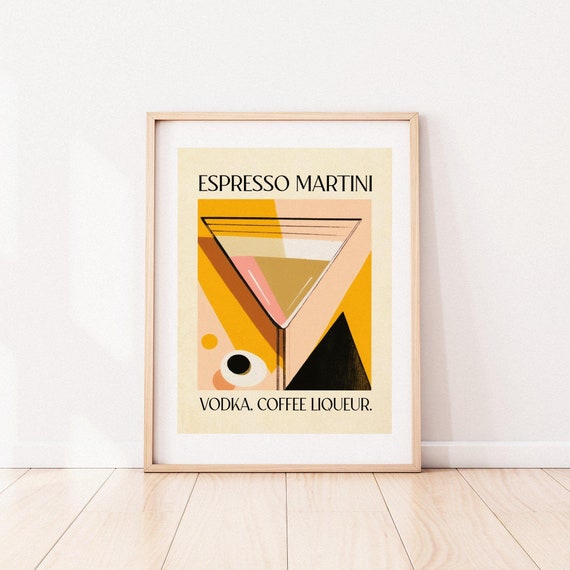This photograph captures a minimalistic and contemporary artwork leaning against a softly painted pinkish-peach wall, which features a white border trim at its base. Below the trim, the floor is composed of wide, shiny, wooden slats that have a subtle peachy hue, indicating a recent waxing. The artwork itself is set in a thin pink frame that complements the gentle tones of the background. Inside the frame, the artwork has a white border and prominently displays the phrases "Espresso Martini" and "Vodka Coffee Liqueur." The central image is a graphic, geometric representation of a martini glass created with a palette of whites, pinks, greens, yellows, blacks, and peaches, giving it a clean, colorful, and modern aesthetic. The piece appears almost like a stylish poster, propped casually against the wall, adding an air of understated elegance to the scene.